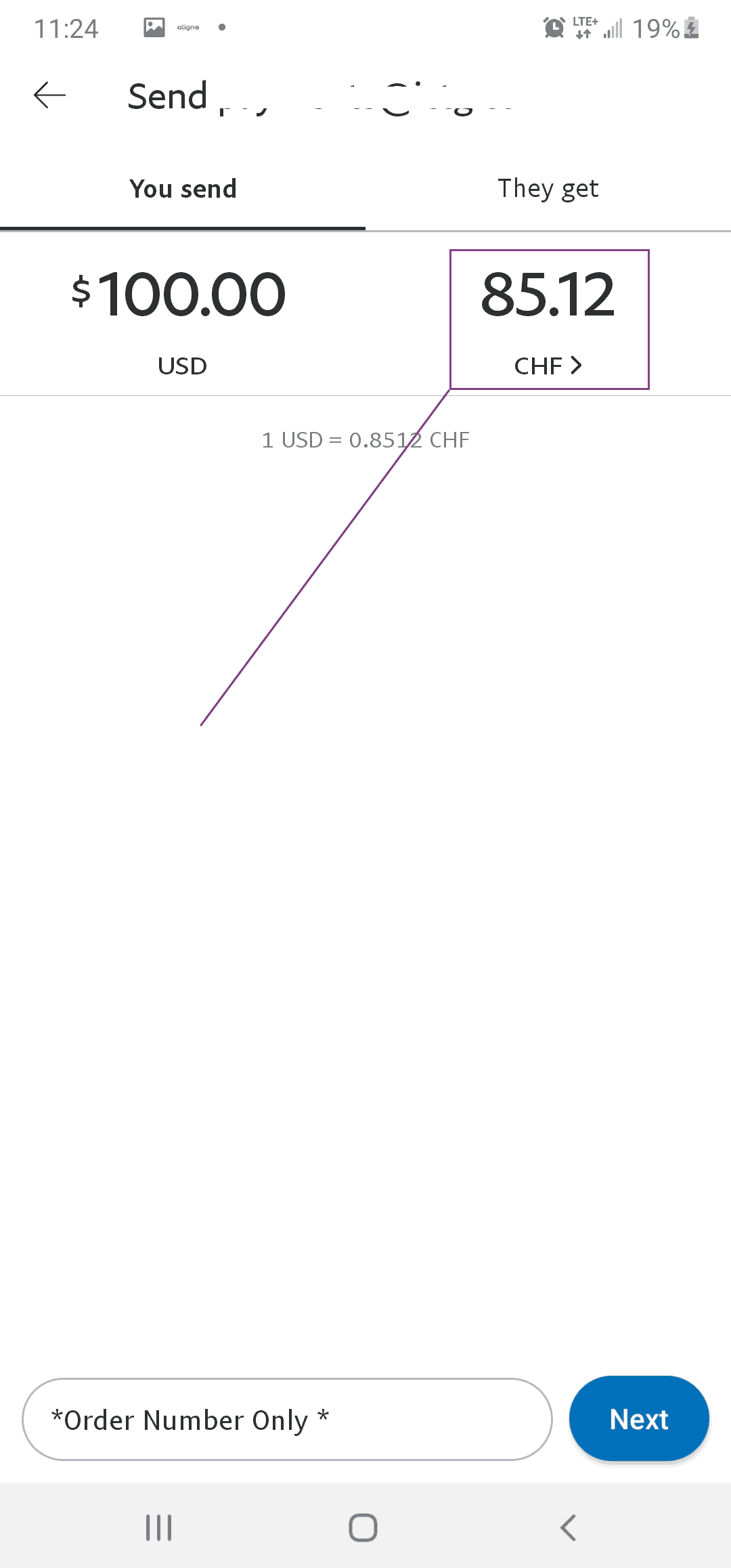**Image Caption:**

The image displays a mobile phone screen with various details visible. At the top right corner, it shows a clock indicating the time as 11:00 and the battery level at 19%. The network status indicates a 4G connection with 'FTE' symbol next to it. An arrow pointing to the left is present on the top left corner, suggesting a 'back' function.

The main content features a transactional interface. It shows the exchange rate, stating that sending 100 US dollars results in receiving 85.12 Swiss Francs (CHF), with an indicated exchange rate of 1 US dollar to 0.85 CHF.

Below this information, there is a text field for the order number, flanked by asterisks on either side. The interface also includes a circular loading or processing icon. A prominent blue button labeled 'Next' is visible towards the bottom of the screen.

Additionally, there is a navigational bar at the bottom of the screen. On the left, it features three vertical lines (hamburger menu icon), a square icon in the center, and a right-pointing chevron (greater than symbol) placed on the right side. The interface also includes a progress line that extends to the right, ending near the CHF amount.

Overall, the image illustrates a detailed screen layout for a financial transaction or money transfer application on a mobile device, providing rich information and user interface elements.